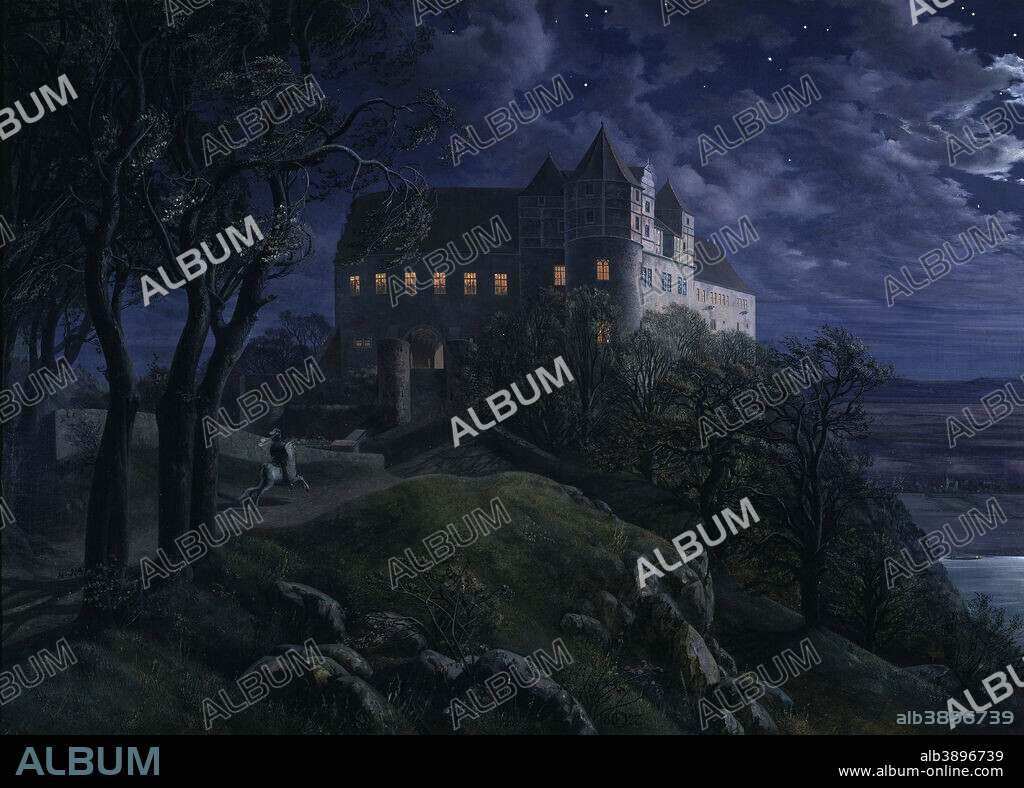The image portrays a detailed painting of a large, castle-like mansion situated atop a hill. The building has a cream-colored exterior and features numerous windows from which warm, yellow light emanates, suggesting an inhabited structure. One corner of the mansion is characterized by a round tower. The surroundings include uneven ground covered in green grass, plants, and rocks, contributing to a rugged terrain. A white horse, ridden by a person, is ascending a trail toward the building, adding to the dynamic sense of the scene. The sky above is a deep, midnight blue, filled with dark, rolling clouds, enhancing the atmosphere with a sense of mystery and unease. The overall scene is dimly lit, suggesting twilight or nighttime. The image is marked by watermarks reading "ALBUM" in a clear, diagonal white outline. At the bottom, a black horizontal strip along the base of the image displays the text "ALBUM" on the left and "ALB3896739 www.album-online.com" on the right.